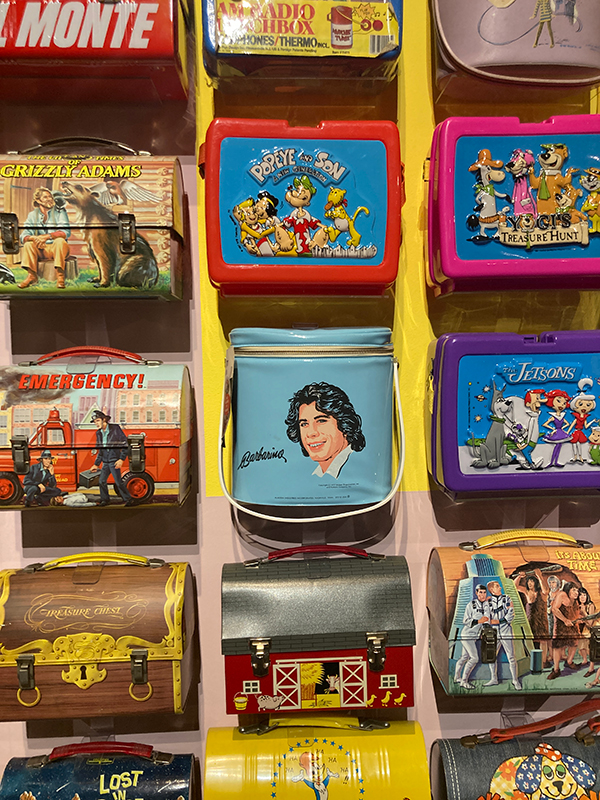This photograph showcases an array of vintage lunchboxes artfully displayed on a wall, organized in rows. Starting from the top left, there's a partially visible lunchbox with "Monte" in white letters on a red background. Below it hangs a Grizzly Adams-themed lunchbox featuring an image of Grizzly Adams accompanied by his bear, with the name "Grizzly Adams" in bold yellow capital letters.

Directly beneath it is a lunchbox depicting a firetruck responding to an emergency, with firefighters and buildings in the background. Next in line is a wooden-themed lunchbox labeled "Treasure Chest," adorned in shades of yellow and brown.

Moving to the middle row, the first lunchbox is unreadable, but the second clearly displays "Popeye and Son," showcasing characters like Popeye, Olive Oyl, and Jeep. Adjacent to it, prominently placed in the center of the image, is a light blue vinyl bucket lunchbox with a white handle underneath, featuring an image of John Travolta from "Saturday Night Fever." To its right is a purple plastic lunchbox decorated with characters from "The Jetsons."

On the top right, a partially visible lunchbox shines with its silver top, and next in the sequence is a hot pink lunchbox featuring characters from the Yogi Bear series, including Quick Draw McGraw, Snagglepuss, Yogi Bear, Boo Boo, and the title "Yogi's Treasure Hunt."

In the bottom row, there’s a distinct purple lunchbox conveying the futuristic flair of "The Jetsons," and the final legible one in this intricate display appears to be a lunchbox labeled "It's About Time," portraying a mix of cavemen and space people, with some uncertainty regarding its exact depiction.